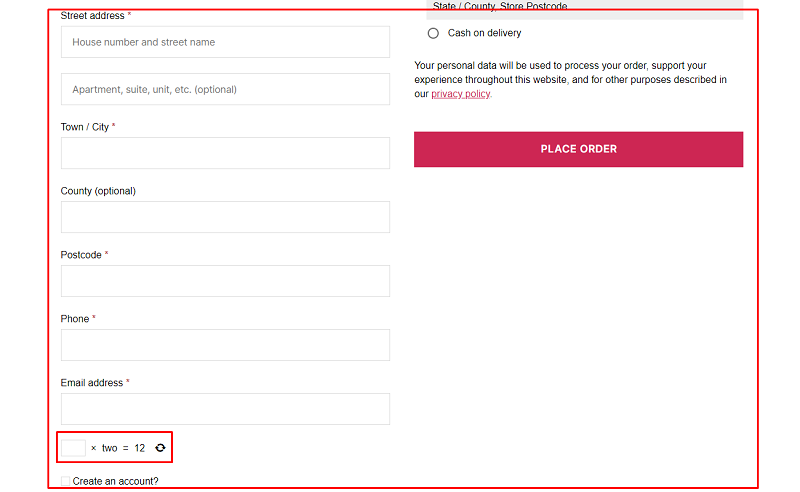This screenshot depicts an online checkout page, bordered by a red outline. The interface appears to be in the process of collecting user information for a potential purchase. At the very top left of the screen, it prompts the user to input their street address. There are six text boxes provided for entering the house number and street name, with optional fields for apartment, suite, or unit numbers. Following this, the page asks for the town or city, again with six text boxes. The county is listed as optional with its own text box.

Further down, the page requests a postcode, a phone number, and an email address, each with designated text boxes. Notably, there is a section towards the bottom with an empty text box accompanied by the equation "times two equals twelve" and a small refresh button, all highlighted by a secondary red outline.

At the very bottom of the screenshot, two buttons are prominently displayed: one labeled "Create Account" and another labeled "Cash on Delivery," which implies an available payment option. The page ultimately leads to a "Place Your Order" button, positioned to the right.